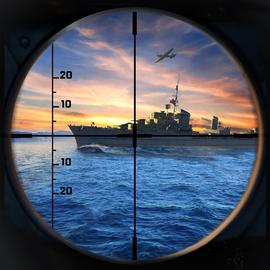This detailed image appears to be a telescopic view, likely from a video game simulating a submarine's perspective as it sights a gray battleship with a blue, choppy ocean as a backdrop. Through the circular lens, the scene is rendered with black corners framing the visuals. The sky blends hues of blue, orange, pink, and yellow, suggesting a sunset or sunrise, accented by dark clouds. A gray airplane flies above the ship. The display includes intersecting black lines: a line bisecting the image vertically and another horizontally, while a numbered scale from 20 to 10 and back to 20 runs along the left side. The numbers and lines, characteristic of a targeting reticle, enhance the tactical appearance of the view.